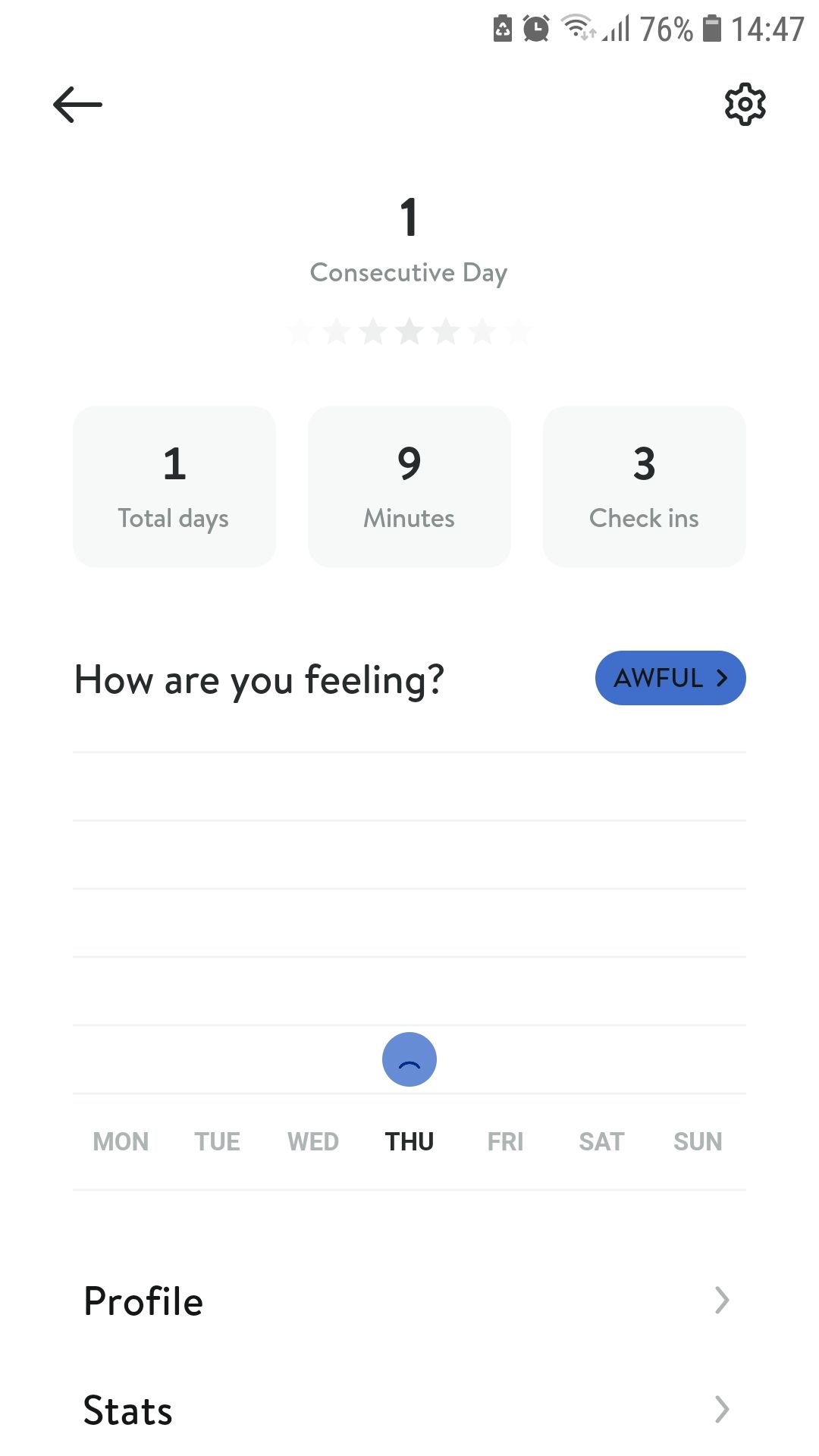A detailed image description of a cell phone screen showing an emotion-tracking app, with intricate interface details:

The image displays a cell phone screen showcasing a page from an emotion-tracking app. At the top of the screen, there is a navigational left arrow, indicating there is a previous page. The upper right corner contains the phone's status icons: the current time, battery percentage, a battery icon, Wi-Fi signal strength, and an alarm clock icon, suggesting that an alarm is set.

Below these icons, a bold black numeral "1" is prominently displayed, followed by the phrase "consecutive days" in gray letters. Beneath this, five star icons are lined up, all grayed out, signifying that none have been selected. Below the stars, there are three horizontally aligned rectangular boxes, each separated by small spaces. The boxes are off-white in color. The first box on the left reads "1 total days," the middle box indicates "9 minutes," and the box on the right states "3 check-ins."

Further down, in solid black text, the app poses the question, "How are you feeling?" Adjacent to this question is a blue button featuring the word "awful" in black letters. To the right of this button, an arrow suggests there are additional options to select from.

The lower portion of the screen presents a day chart spanning Monday through Sunday. A small, frowning circle icon, indicating a negative emotion, is positioned over Thursday in the middle of the chart. Beneath this chart, there are two options labeled "Profile" and "Stats," each accompanied by a right arrow icon, hinting at the ability to navigate to these pages.